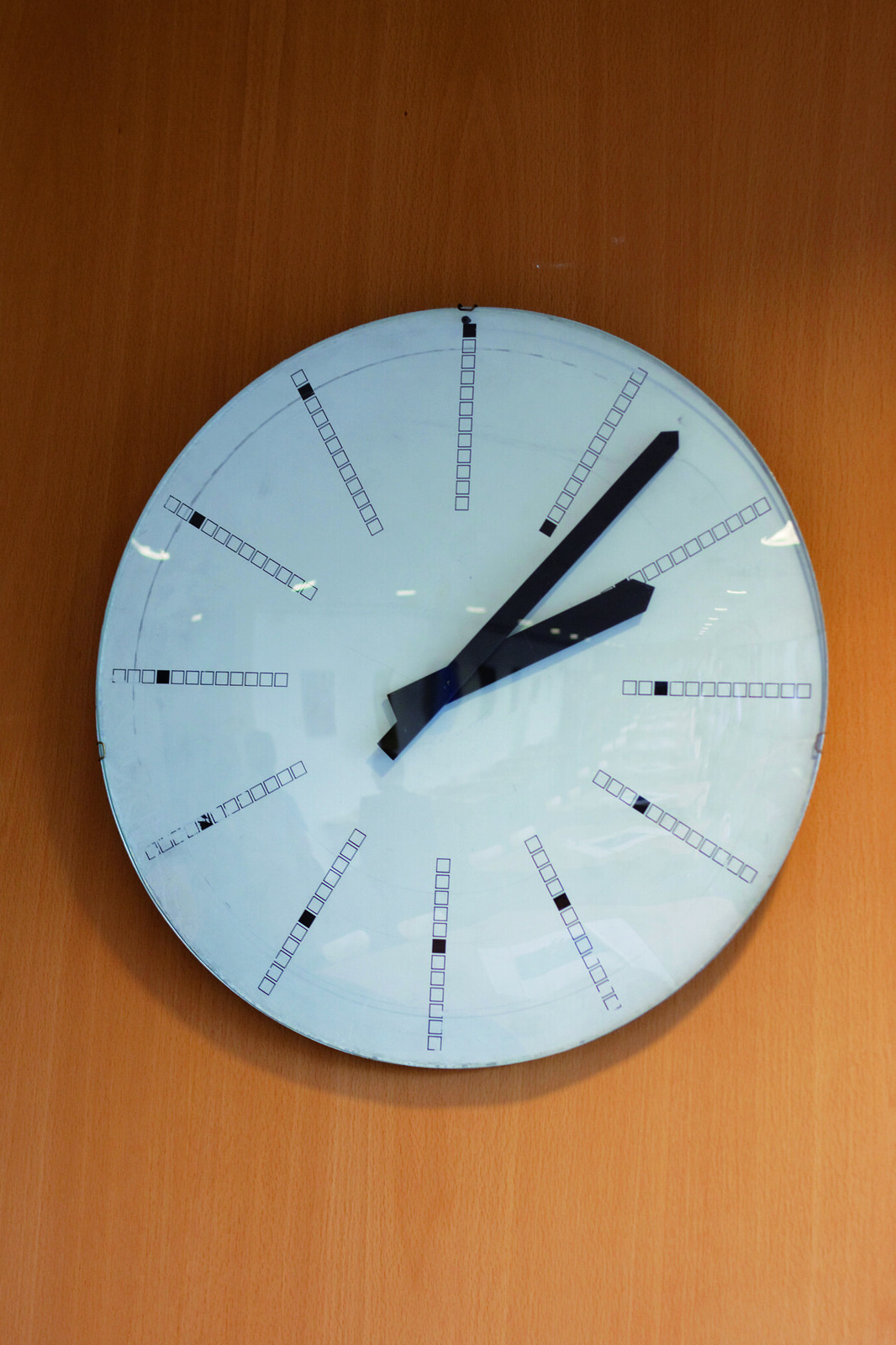The image showcases a large, circular clock hanging on a vertically-lined, orange-brown wooden wall. Instead of traditional numbers or Roman numerals, the clock features a series of 12 squares arranged along its perimeter to represent the hours. Each number is indicated by a blackened square within this line of squares: the first square is black for 1 o'clock, the second square is black for 2 o'clock, and this pattern continues until the 12th square is black for 12 o'clock. The face of the clock is white, and it has sleek black hands indicating that the time is approximately 2:07. The clock appears to have a glass surface, reflecting what seems like a classroom environment.